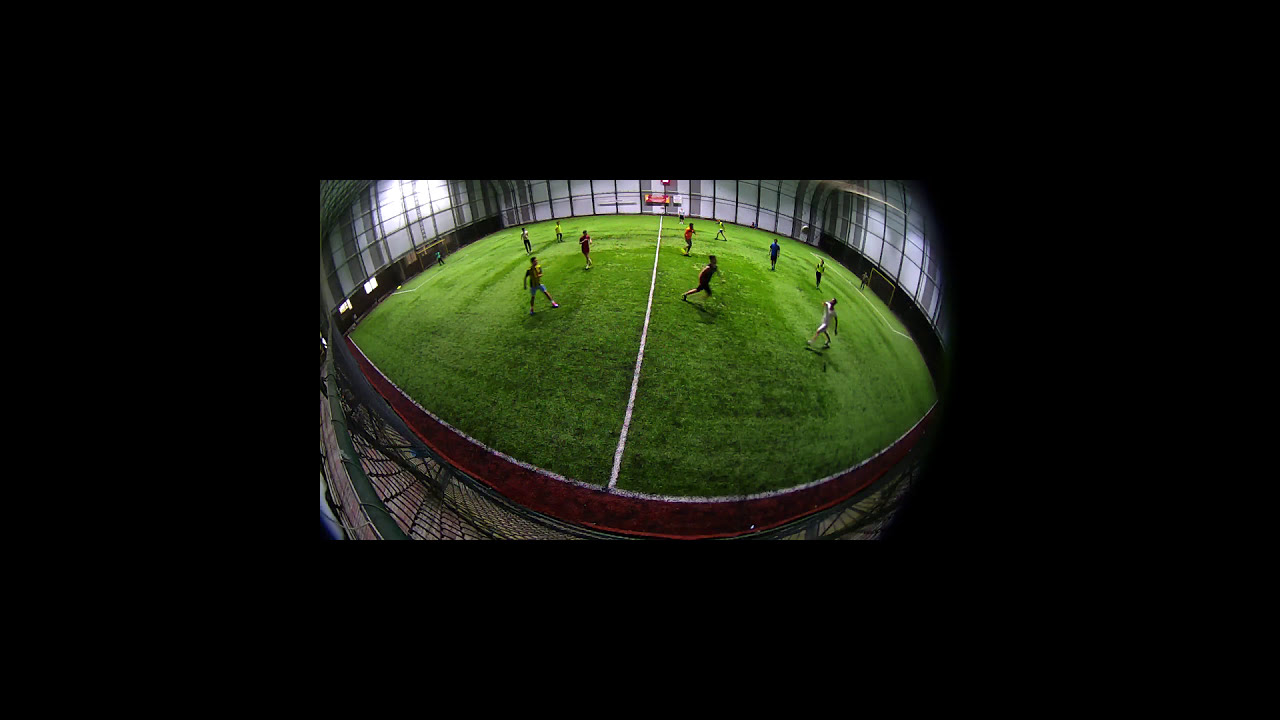The photograph captures an indoor soccer game from a top-down perspective, likely distorted by a fisheye lens. The field is smaller than a professional one, encased within a thick black border that frames the image. The lush, vibrant green field is distinctly marked with white lines down the center, along the edges, and around the goals, delineating the areas of play. Rectangular white goalposts adorned with nets stand on either side, guarded by goalies. Approximately 11 to 12 active players, whose identities are indistinguishable due to the distance, populate the field. The far wall of the arena is a steel gray, while artificial lighting emanates from the top and the walls behind the goalposts. The image has a somewhat abstract, curved appearance, contributing to the illusion of an oval-shaped field. A faint scoreboard is visible in the background, adding to the scene's lively yet focused ambiance.